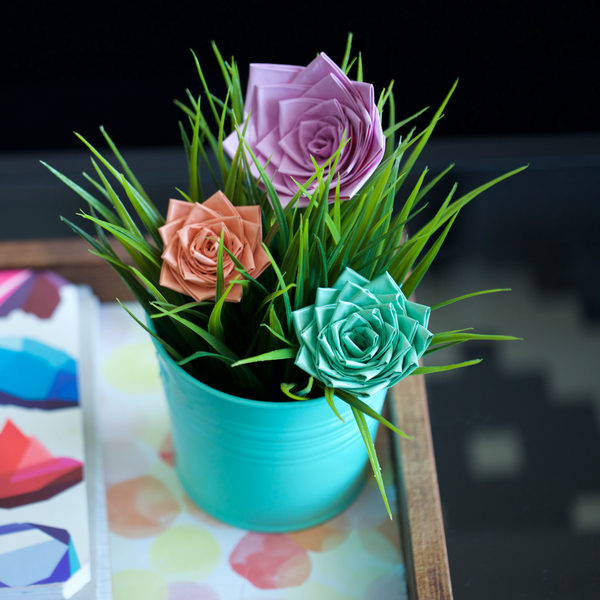In an indoor setting, a pale light blue metal pot sits on a table adorned with a vibrant, multi-colored tablecloth that features a mix of purple, blue, red, and white shapes. The table itself is bordered by a brown wooden berm. Inside the pot, there are three delicate paper flowers of different colors: a teal blue flower positioned at the lower right, a peach flower to the upper left, and a larger purple or lavender flower at the top. These flowers are surrounded by deep green foliage resembling palm leaves, adding a lush contrast. The background behind and to the sides of the pot is gray, while the area beneath the table appears to have a blue carpet. Scattered papers and watercolor-like art supplies are also visible on the table, enhancing the creative atmosphere of the scene.